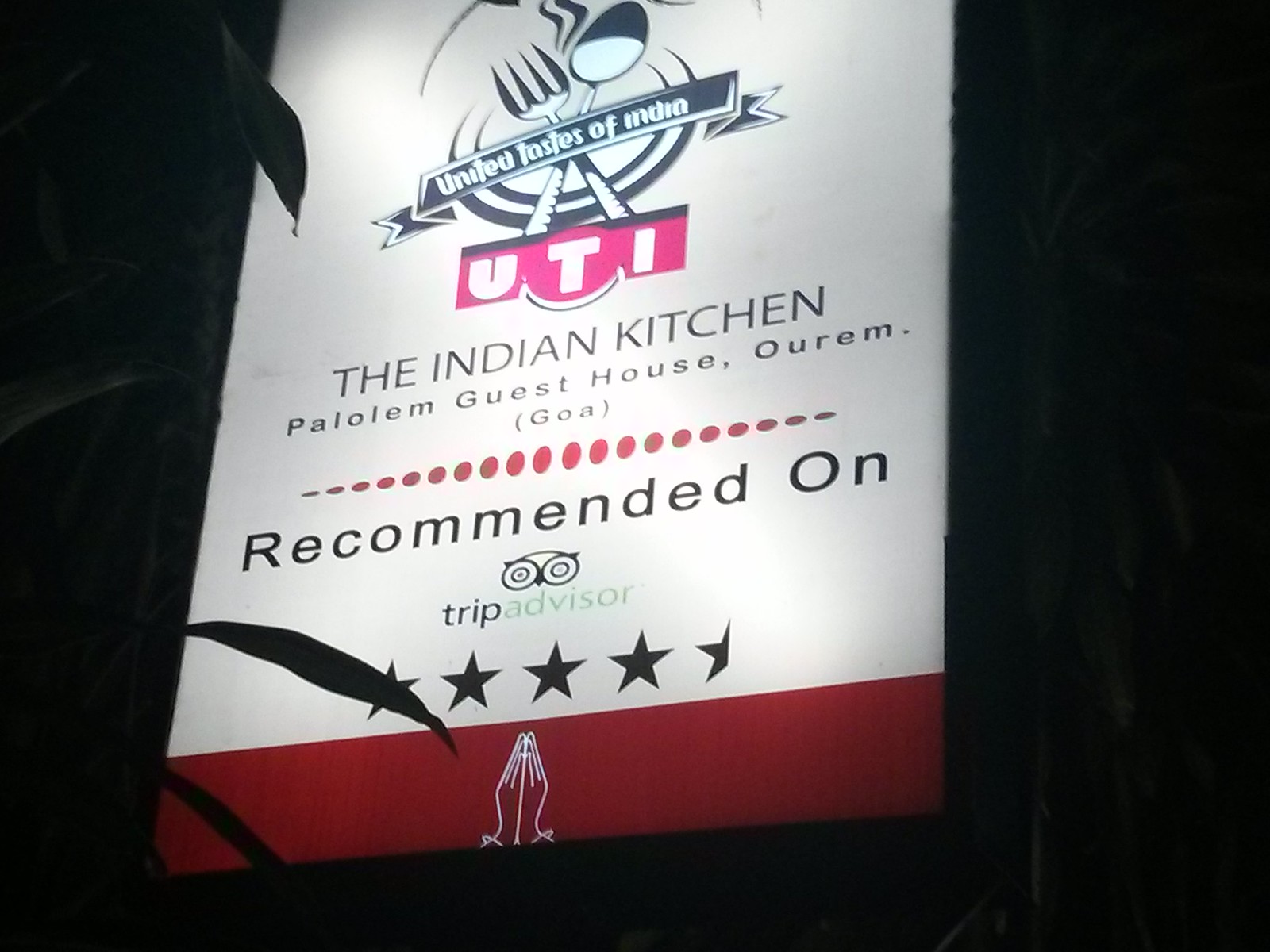The photograph captures a large, illuminated sign taken at night, showcasing an advertisement for a restaurant called "United Taste of India" (UTI). The sign predominantly features a light-colored background with silhouetted tree branches, suggesting an outdoor setting. At the top of the sign, a black and white graphic of a plate flanked by a spoon and fork is prominently displayed, accompanied by a banner reading "United Taste of India."

Beneath this, a bold red rectangle features the white letters "UTI." Below it, in black text, the sign lists "The Indian Kitchen, P-A-L-O-L-E-M Guest House, O-U-R-E-M (GOA)." A series of red circles two-thirds down the sign denote a boundary, followed by the text "Recommended on TripAdvisor" in black, accompanied by the TripAdvisor owl logo and a rating of four and a half stars. The entirety of the image is framed by the inky darkness of the night, with visible palm trees flanking the sign on either side.